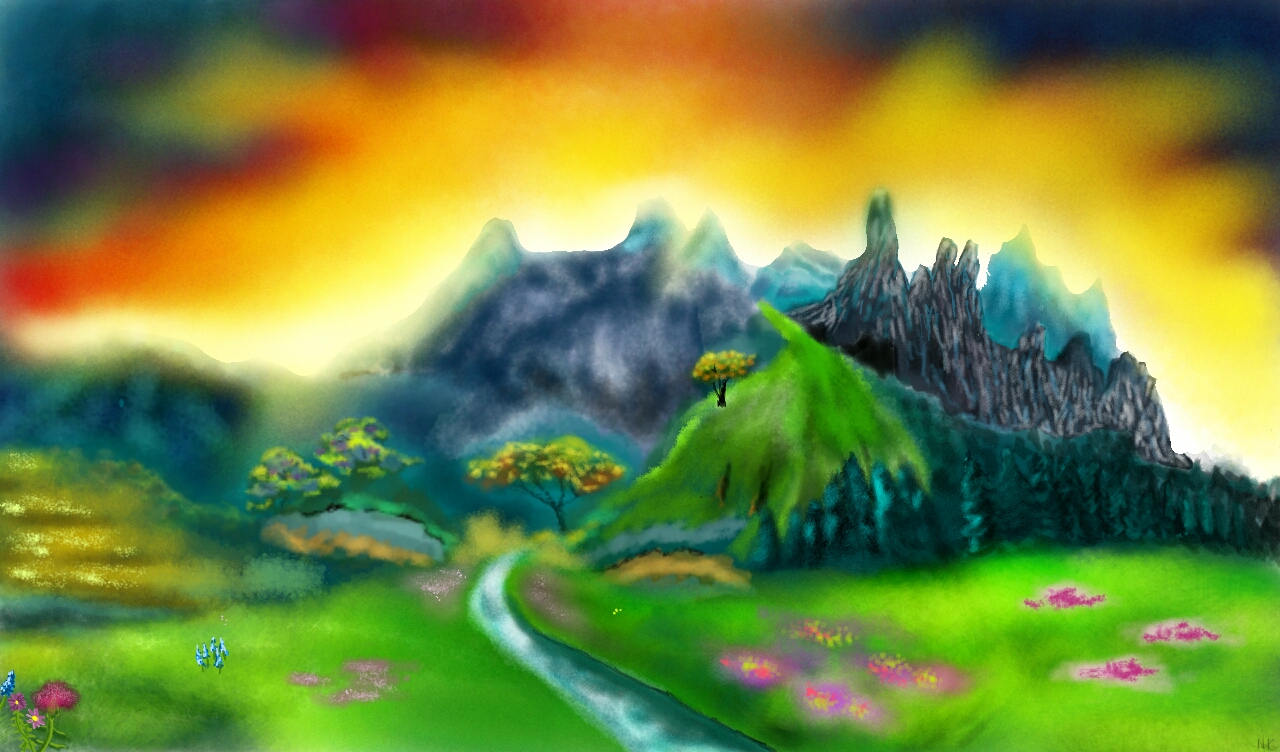In this horizontally oriented rectangular artwork, the scene captures the essence of a magical, fantasy realm. The lush green valley at the forefront is bisected by a meandering river that flows from the bottom center of the image towards a majestic mountain range in the distance. The mountains to the left, painted in muted shades of gray and green, have blurred, jagged peaks, creating a sense of depth and distance. In contrast, the mountains on the right are rendered in sharper, more vibrant hues of gray and black, adding a striking variation to the landscape.

The valley floor is a rich carpet of green grass interspersed with patches of vibrant pink and yellow flowers, adding bursts of color to the scene. A separate field of yellow flowers or grass is visible in the upper left section of the artwork, enhancing the idyllic pastoral atmosphere. In the lower left corner, miniature blue and white figures can be seen, possibly representing people, adding a sense of scale and activity to the serene environment. The ambiguity of their form—whether heads, legs, or merely diminutive silhouettes—adds an element of mystery to this enchanting tableau.